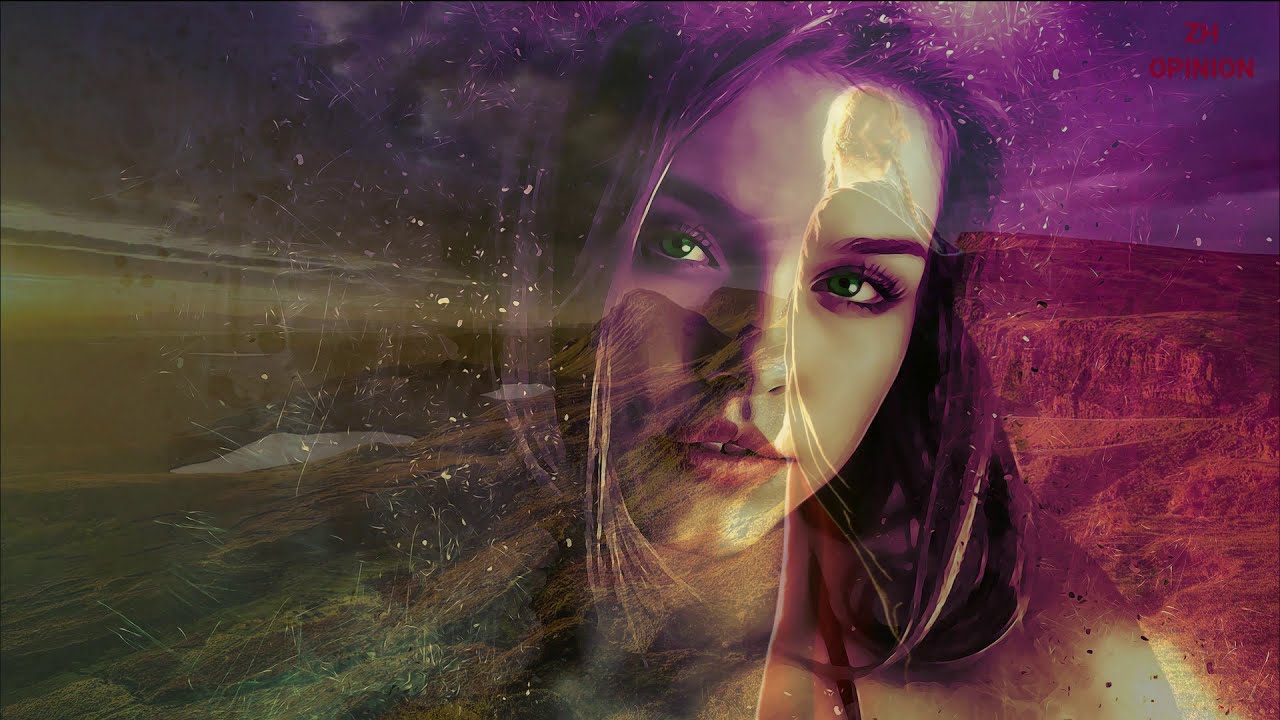A detailed image description:

The image depicts a young Caucasian woman in her late teens to early twenties, with vivid green eyes and light-colored, shoulder-length hair that transitions from brown or dark reddish on one side to purplish and red hues on the other. Her hair appears partially blonde towards the bottom left corner, merging with elements resembling ocean water. She has a serious, almost arresting gaze, clear smooth skin, and red lips, and wears either a black or red halter top with a string around her neck. 

Superimposed and semi-transparent elements overlay her face: on the right, a young girl with blonde hair in pigtails wearing a cloak is positioned, giving the impression she is in the woman's mind. The background to the left is digitally altered, showing a cosmic scene of black with white dots surrounding a cotton ball-shaped creature with tentacles. To the right, the background showcases a purplish-brown hue resembling the Grand Canyon under a purple sky.

In the upper right corner, there's red text reading "Z.H. Opinion," adding an editorial touch to the scene. The blending of multiple elements and themes – cosmic, oceanic, and canyon landscapes – creates a multifaceted and vivid image.